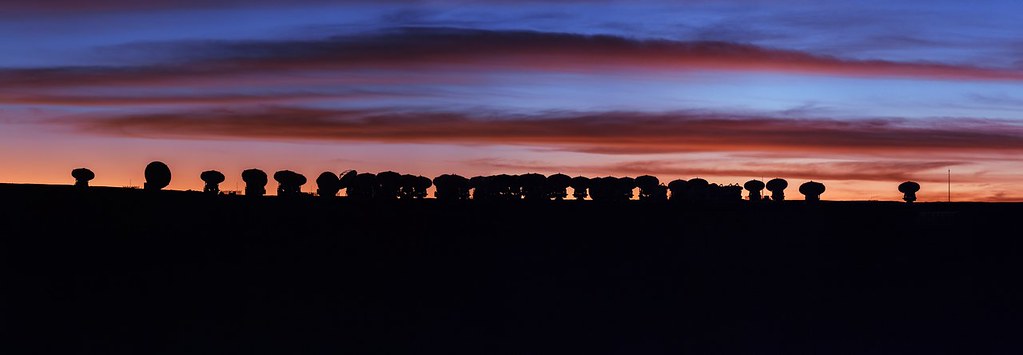The image is a horizontally rectangular outdoor photograph taken during either sunset or sunrise, with no distinctive border or background. The lower third of the image is enveloped in blackness, showcasing the dark silhouettes of trees, which some might mistake for mushroom shapes. A potential power line pole is noticeable on the far center right, rising into the sky. The sky itself is a gradient masterpiece, beginning with hues of orange, red, and pink near the horizon that gradually transition into a dark blue further up. Parallel, ominous clouds stretch horizontally across the sky, tinged with fuchsia and creating a stark contrast with the deepening blue. The ground is completely dark, providing an uninterrupted silhouetted horizon where various indistinct shapes, possibly satellite dishes, stand against the colorful backdrop.